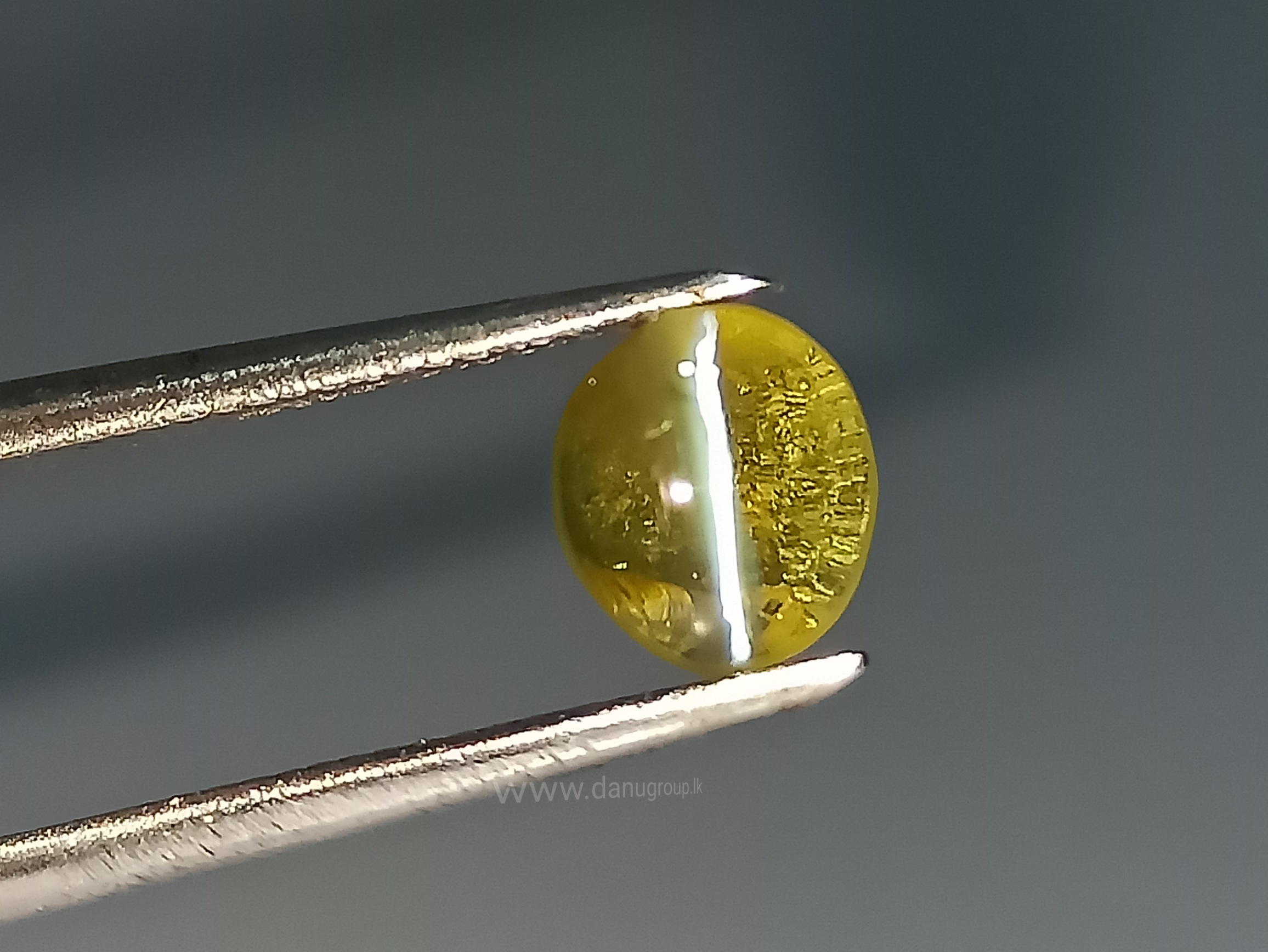In this detailed photograph, a pair of shiny, silver tweezers holds a small, gold-colored stone with a crystallized, semi-transparent appearance. The stone, which is oval in shape, features a distinct white stripe running down its length and catches a reflective light that highlights its lustrous surface. Central to the composition, the stone is meticulously positioned between the tweezers and stands out starkly against the plain gray background. The image is rectangular and horizontally oriented, enclosing the subject within a tidy 5x5 frame. Notably, the image includes a web address, www.danugroup.lk, suggesting it might be a snapshot from a website. However, no additional details such as the photographer, the exact type of stone, the date, or the origin are provided. The overall aesthetic is clean and professional, focusing purely on showcasing the intriguing, gem-like quality of the stone.